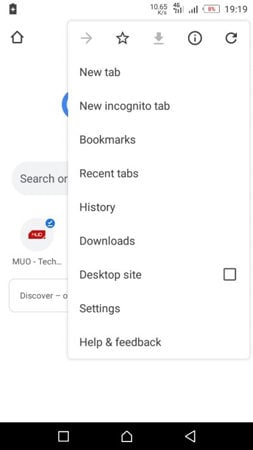This image depicts a blurry, low-resolution screen on an unidentified device. Despite the poor image quality, several details are discernible. 

In the upper left corner, there is a battery icon that indicates charging. Adjacent to it on the right, the screen displays "10.65 k/m," followed by a series of icons. To the right of this text is a cellular icon, further right is another battery icon, and finally, the time is shown as "19:19."

Just below this top row, there are additional icons lined up from left to right: a forward arrow (likely representing a 'next' function), a bookmark symbol, a download icon, an information (i) icon, and a refresh icon.

The lower section of the screen is populated with a list of tabs and menu options, organized vertically. These read from top to bottom as follows: "New tab," "New incognito tab," "Bookmarks," "Recent tabs," "History," "Downloads," and "Desktop."

Overall, the image attempts to convey the interface and functionalities available on this particular device screen, though the clarity is notably compromised.